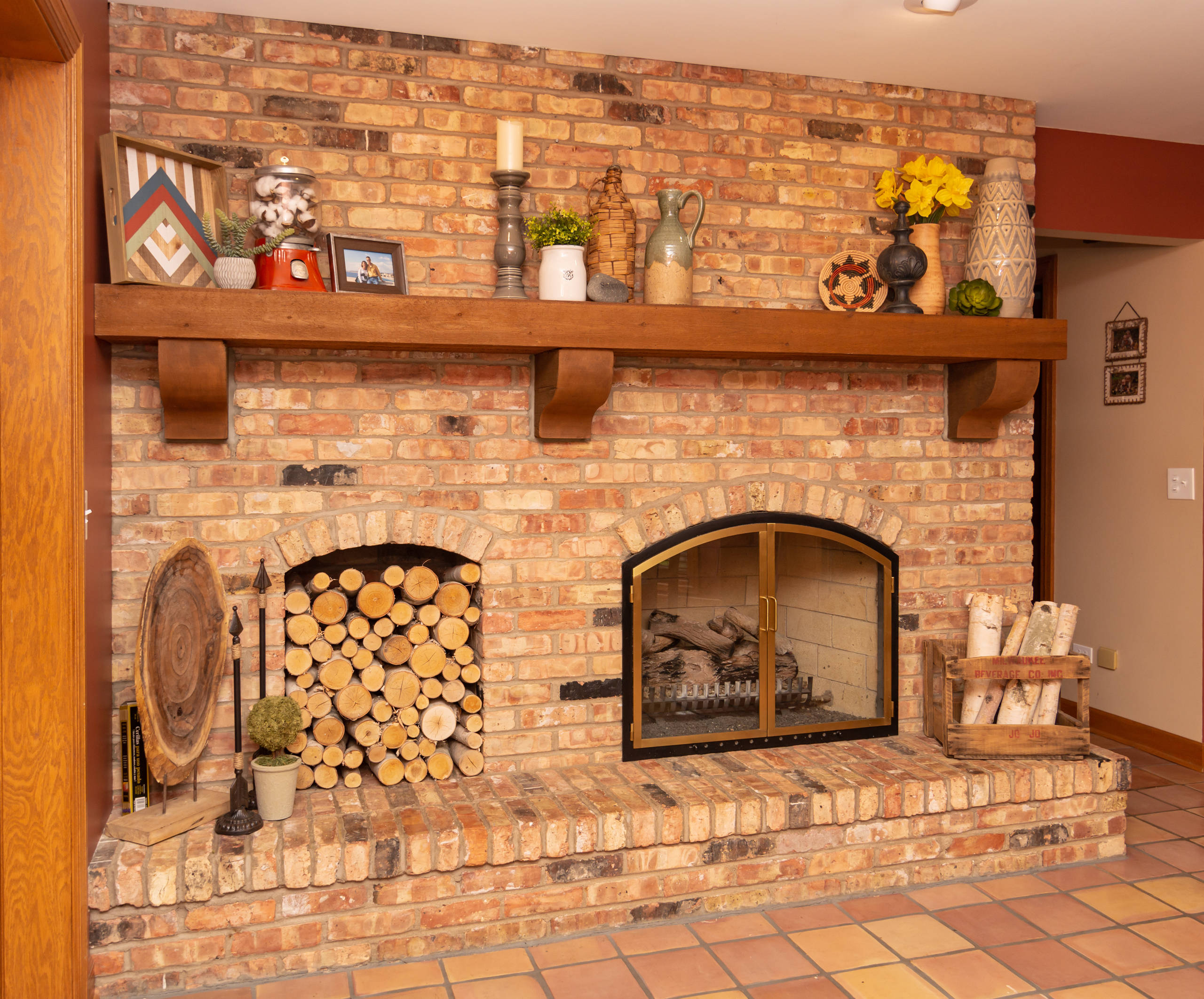This indoor color photograph showcases a cozy room with a commanding brick fireplace that occupies the majority of one wall. The entire wall is constructed from light red to brown tan brick, extending from the floor to the ceiling. Central to the image is the fireplace with its arched hearth, fitted with glass doors encased in gold and black molding. Inside, a pile of logs awaits ignition on the grate. Adjacent to the fireplace on the right, a wooden crate also holds some logs, ready for use. Notably, there is a generously-sized cutout in the brick wall on the left side, matching the height of the fireplace, filled with neatly stacked firewood. 

A predominant feature is the large wooden mantle above the fireplace, supported by three robust wooden sconces. The mantle is adorned with rustic and local country art, including framed photographs, tall pillar candles, vases with flowers, an old milk jug or water jug, and various handmade wooden objects. The hearth itself is somewhat raised, a tiled step up from the floor. The flooring in front of the fireplace consists of orange square terracotta tiles, lending warmth and contrast to the earthy brick and rustic decor. 

In addition, the right side of the image reveals a hallway leading to another room, where white walls, wooden baseboards, and a wooden beam cornice are visible, adorned with two small, vertically-stacked framed photographs. The overall ambiance of the room is one of warmth and rustic charm, with each decorative detail contributing to a cozy, inviting space.